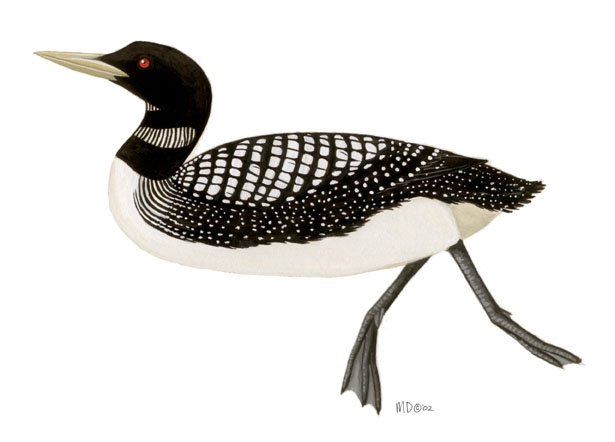This detailed drawing depicts a duck facing towards the left. The duck features a long, beige beak with accents of olive green and light brown, and it has beady, red eyes with black pupils. The head of the duck, encompassing its crown, is jet black. As the neck begins, it displays a unique pattern composed of black and white lines separated by a large black streak that extends from the base of the neck to the back of the head. Further down, there is more black and white lining, intersected by another jet black stripe that wraps around the neck. The underside of the duck is completely white, starting from the jet black stripe at the neck's end. 

The back of the duck showcases a variety of patterns: black and white lines curve towards the right side near the tail, transitioning into a polka-dotted black streak. This dotted pattern gives way to solid jet black feathers towards the end of the tail and along the edges of the wings. The top of the bird's back features a distinctive spiderweb-like pattern, with white feathers adorned by black vertical and horizontal lines where the horizontal ones are thick and vertical ones thin. The legs, positioned in a 'V' shape, are dark gray and webbed, suitable for swimming.

The background is purely white, emphasizing the floating appearance of the duck, which seems to be in mid-motion, as if paddling through water. Below the duck, between its legs and near its right foot, is the artist’s signature in black thin lines, reading “MD © 02.”